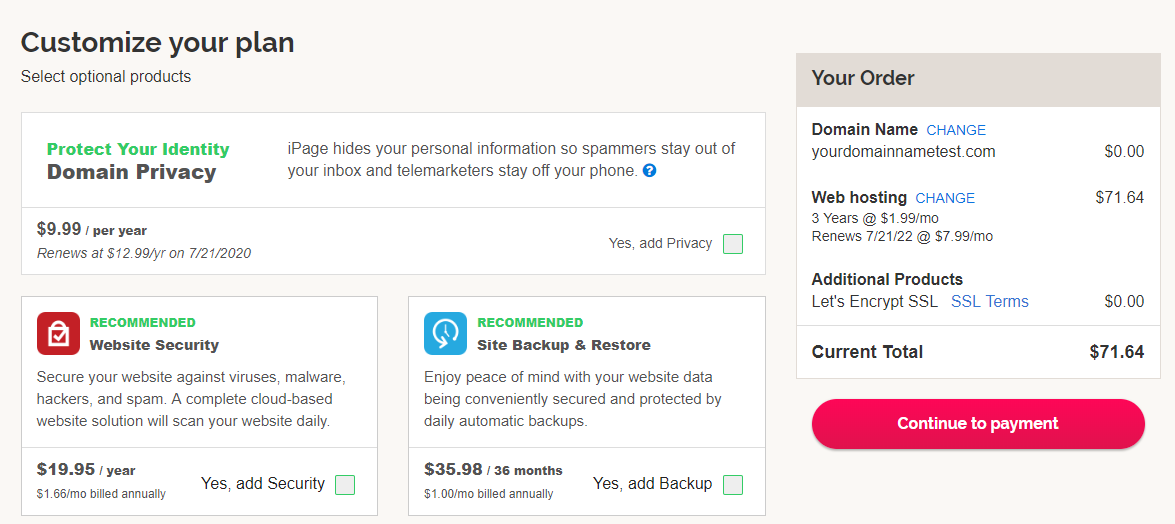The webpage displays a section with a light cream-white background, featuring various customizable options for users to enhance their plans. At the top left, bold black text reads "Customize Your Plan," followed by instructions in smaller black text to "select all the optional products."

1. **Protect Your Identity**:
   - Written in green text for emphasis.
   - Description: "Domain privacy ensures that your personal information is hidden, keeping spammers out of your inbox and telemarketers off your phone."
   - Price: "$9.99 per year, renewing at $12.99 per year starting on 7-21-2020."
   - A checkbox option labeled "Yes, add privacy."

2. **Website Security**:
   - Marked as "Recommended" with the label in green text.
   - Description: "Secure your website against viruses, malware, hackers, and spam with a complete cloud-based solution that scales your website daily."
   - Price: "$19.95 per year, which is $1.66 per month, billed annually."
   - A checkbox option labeled "Yes, add security."

3. **Site Backup and Restore**:
   - Also marked as "Recommended" with the label in green text.
   - Description: "Enjoy peace of mind with your website data being securely backed up by Dell Automatic Backups."
   - Price: "$35.98 for 36 months, which is $1 per month, billed annually."
   - A checkbox option labeled "Yes, add backup."

On the right, the "Your Order" section summarizes the selected options:
- Domain Name: "yourdomainnametest.com"
- Web Hosting and Additional Products
- Current Total: "$71.64"

At the bottom right, a prominent red button labeled "Continue to Payment" encourages users to proceed with their purchase.